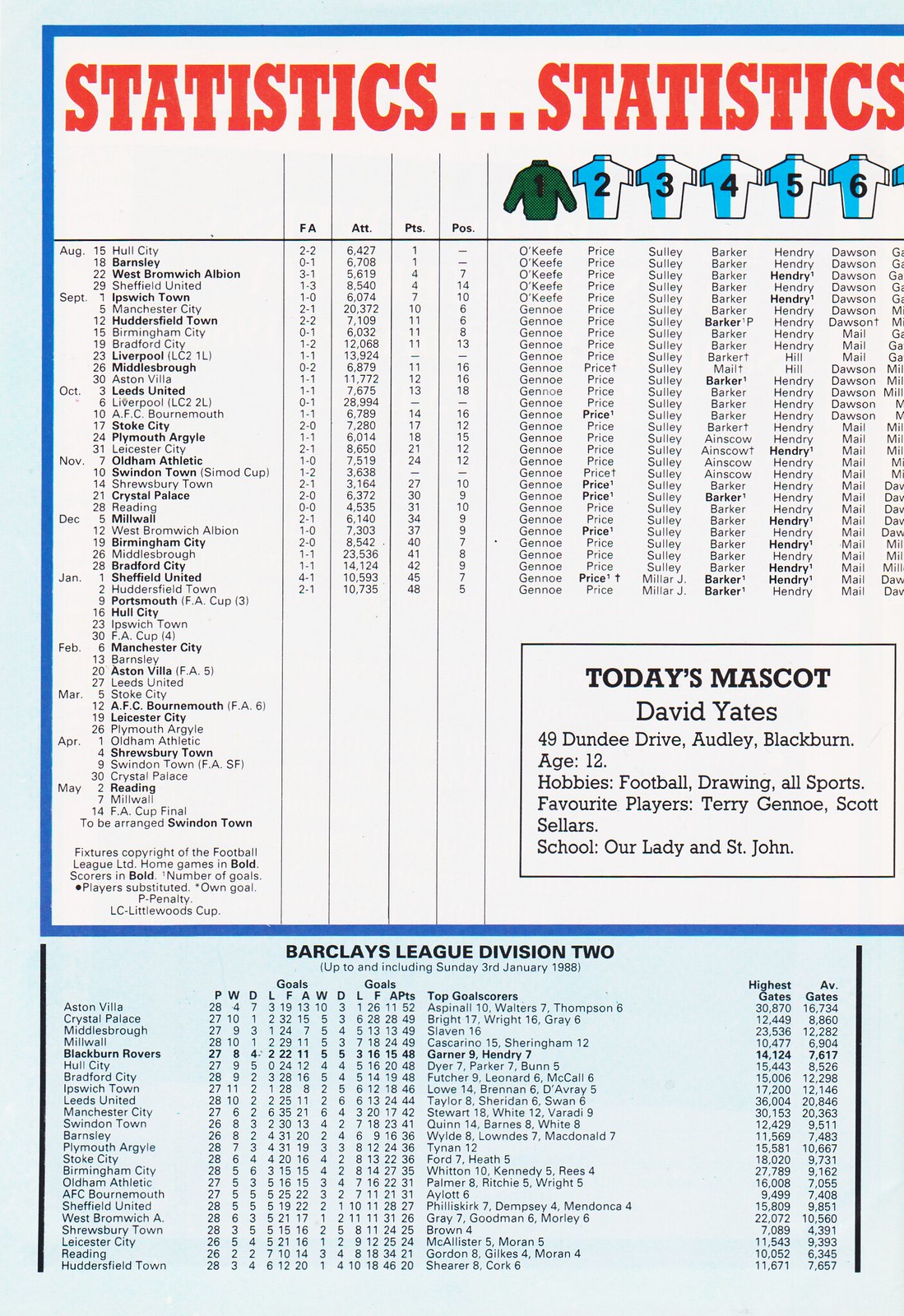The image, likely taken from a magazine, presents detailed match day statistics for the Barclays League Division II. The title at the top of the page reads "Statistics... Statistics" in red text, framed by a blue border. The upper section includes a list of teams along with various statistics, such as points, attempts, attendance numbers (A.T.T.), and positions (P.O.S.), displayed for dates ranging from August through March. In the center, there's a highlighted square introducing "Today's Mascot" - David Yates, age 12, from Dundee Drive, Potlick, Blackburn. It shares details about his hobbies (football, drawing, all sports), favorite players (Terry Gano, Scott Sellers), and school (Our Lady and St John). Near the bottom of the image, standings for the Barclays League Division II teams are listed, with top goal scorers featured on the right. Additionally, six jerseys are shown with corresponding player names, depicting team colors—green, blue on the left, and white on the right.